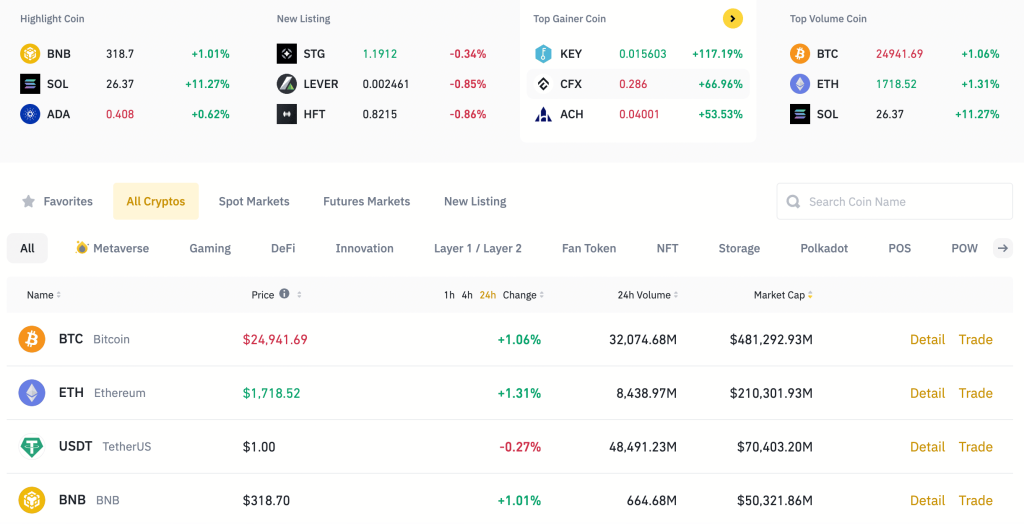This detailed screenshot of cryptocurrency charts exhibits intricate information related to various crypto assets. 

**Top Chart**: 
- **Columns**: The chart is divided into multiple columns, each dedicated to specific information regarding cryptocurrency performance:
  1. **"Highlight Coin"**: Features three prominent cryptocurrencies – BNB (Binance Coin), SOL (Solana), and ADA (Cardano). Displayed alongside these coins are metrics indicating their recent performance, including price increase and trading volume.
  2. **"New Listing"**: Showcases newly listed cryptocurrencies.
  3. **"Top Gainer Coins"**: Identifies the top-performing cryptocurrencies, marked with a yellow circle and a black arrow pointing to the right, signifying upward trends.
  4. **"Top Volume Coin"**: Lists cryptocurrencies with the highest trading volumes.

**Example Data**: 
- For **"Highlight Coin"**, the listed coins (BNB, SOL, ADA) show their updated prices, percentage increase, and trading volumes.

**Second Chart**:
- **Tabs and Search Functionality**: A search bar is positioned in the top right corner for easy navigation. On the left-hand side are five tabs:
  1. **Favorites**
  2. **All Cryptos** (highlighted in yellow)
  3. **Spot Markets**
  4. **Future Markets**
  5. **New Listing**

- **Displayed Data**: Under the "All Cryptos" tab, the chart provides comprehensive data for various cryptocurrencies. Each row includes:
  - **Name**: The acronym for the cryptocurrency (e.g., BTC for Bitcoin, ETH for Ethereum, USDT for Tether US, and BNB).
  - **Price**: Current market price (e.g., Bitcoin is $24,941.61).
  - **Change in 1h, 4h, 24h**: The percentage change over one hour, four hours, and twenty-four hours.
  - **24h Volume**: Trading volume over the past 24 hours (e.g., for Bitcoin, it’s $32,074.68).
  - **Market Cap**: The total market capitalization (e.g., Bitcoin has a market cap of $481,292.93).

- **Additional Features**: Each row includes a "Detail" link and a "Trade" link for further actions.

This well-structured display provides extensive insights into cryptocurrency performance, aiding traders in making informed decisions.